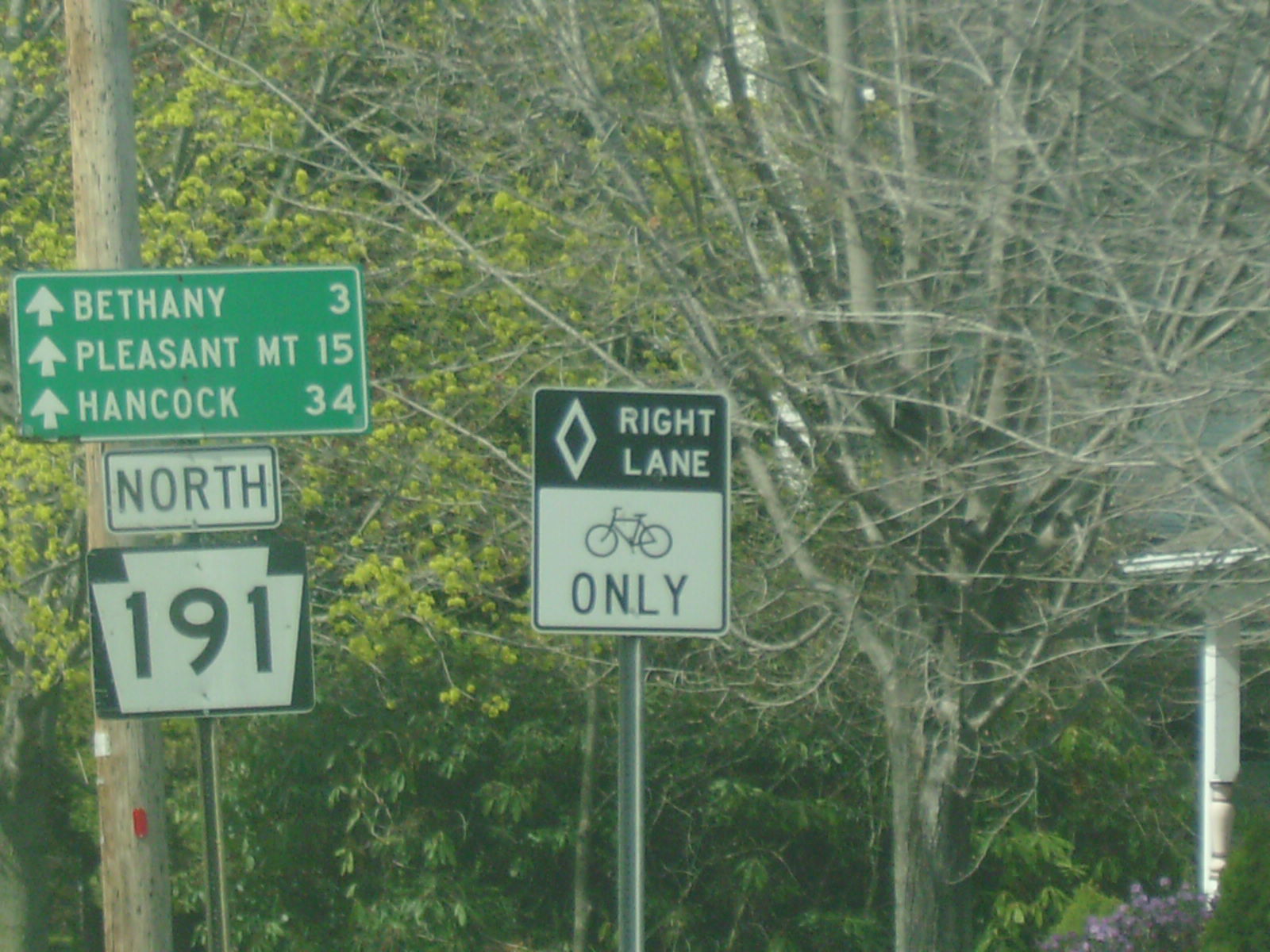The image features an array of highway signs set against a backdrop of tall, verdant trees characterized by a mix of green and bright yellow-green leaves. The primary highway sign is rectangular and green, with crisp white lettering detailing three different destinations, each accompanied by an upward-pointing white arrow indicating they are straight ahead. The first destination, "Bethany," is listed as being 3 miles away. The second, "Pleasant Mountain," is 15 miles distant, and the third, "Hancock," is 34 miles away. Below this main sign, there's an additional sign displaying "North," and beneath that, a smaller sign marked "191." These signs are framed by the vibrant foliage, which adds a lively and natural background to the scene.